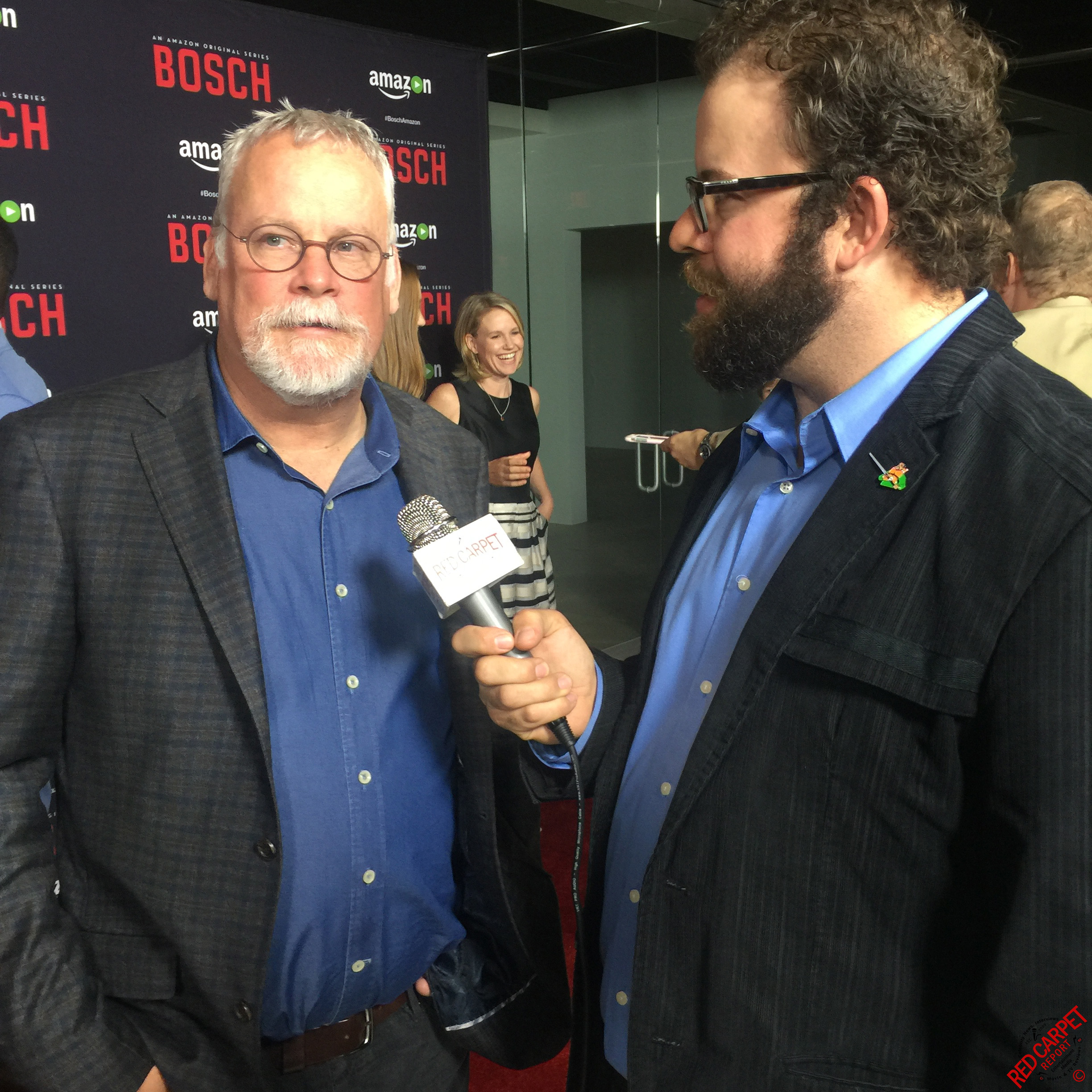This image captures a red carpet interview at a premiere event for an Amazon show called Bosch. The focus is on two gentlemen standing in the foreground. The interviewer, positioned on the right, is a man with short, curly, blonde-brown hair, a brown beard, and black rimmed glasses. He is dressed in a dark navy blue, pinstripe jacket with a small colorful pin on the lapel, a blue button-down shirt underneath, and he holds a microphone with a white sign on it. The interviewee, on the left, has short, straight gray hair, a gray beard, round reddish glasses, and is wearing a dark gray plaid blazer over a blue button-down shirt. Around them, other attendees are visible, engaging in conversation and interacting against a backdrop that features sponsor logos including Bosch in red letters and the Amazon Prime logo. The bottom right corner of the image subtly reveals the words "red carpet" in small red letters, further emphasizing the event setting.